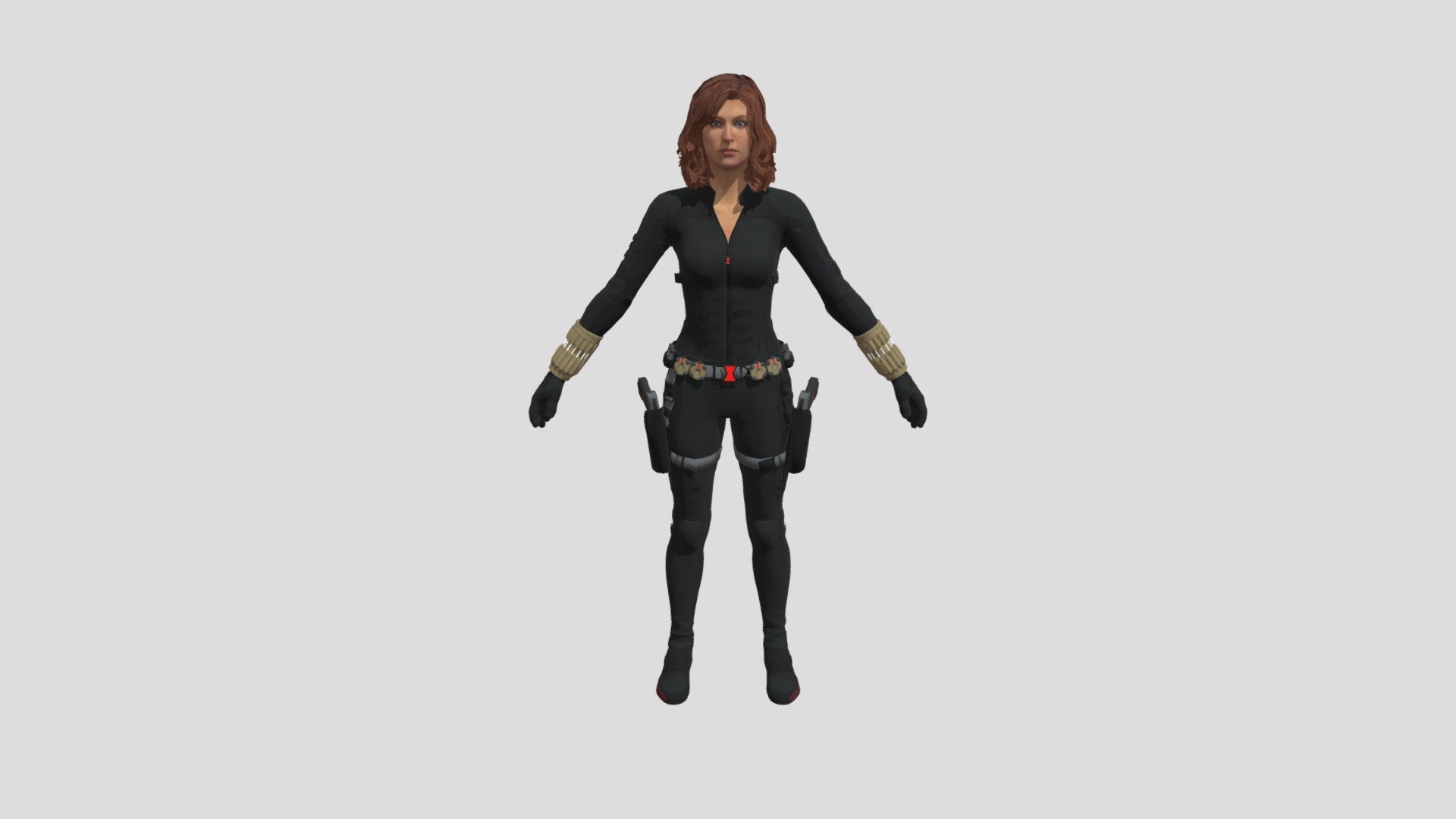The image depicts a detailed 3D model of a female video game character. She is positioned at the center of a wide horizontal frame with a light gray background. The character has light pinkish skin and a stern expression. Her light brown, wavy hair falls just above her shoulders. She is clad in a charcoal gray, long-sleeved bodysuit featuring a V-neck and collar. The bodysuit extends down to her legs, which are slightly apart. Over the bodysuit, she wears black boots that reach up to her thighs.

Her attire includes light gray wristbands and a utility belt around her waist, equipped with various items in shades of gray, red, and blue. Her wrists are also adorned with gray cuff-like accessories, and she is wearing black rubber gloves. Each thigh has a gun holster strapped to it, each containing a firearm. The character stands with her arms angled slightly down and away from her sides, staring directly at the camera, which enhances the image's sense of realism and depth.